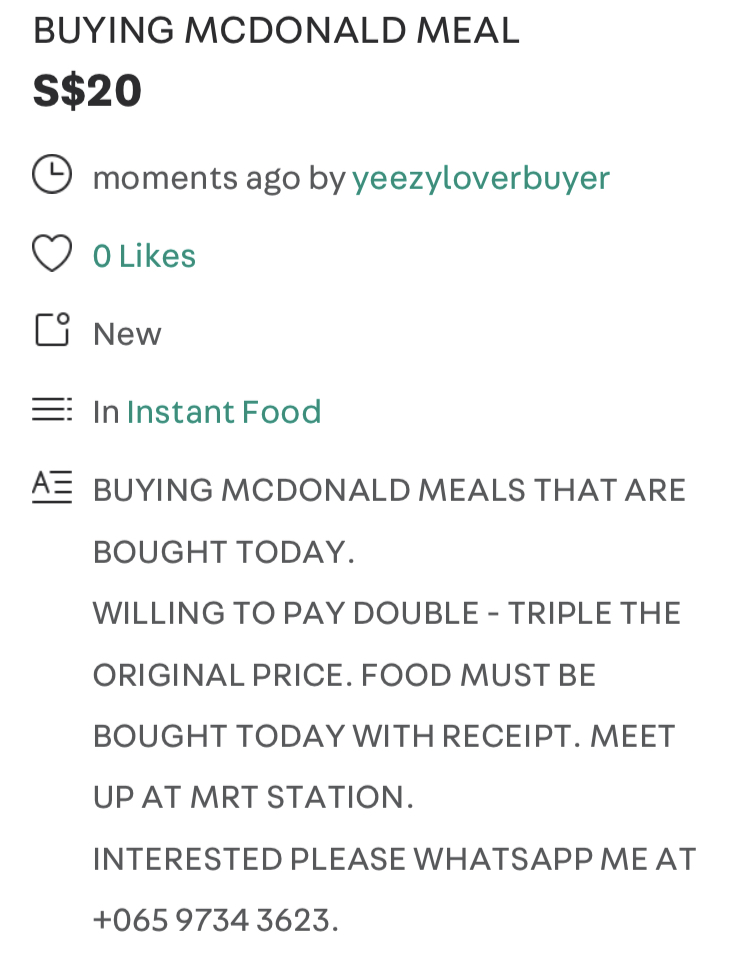This image showcases a listing for purchasing McDonald's meals. It prominently displays a headline reading "Buying McDonald's Meal" with a price of $20. The post was made a few moments ago by a user named "easy lover buyer" and currently has zero likes. The post is tagged as "new" and categorized under "Instant Food."

Further details at the bottom mention the buyer's willingness to pay double or triple the original price for McDonald's meals that must be bought on the same day and accompanied by receipts. The specified meetup location is Miss March station. Interested parties are requested to contact the buyer via WhatsApp at +06 59 7 3 4 3 6 2 3.